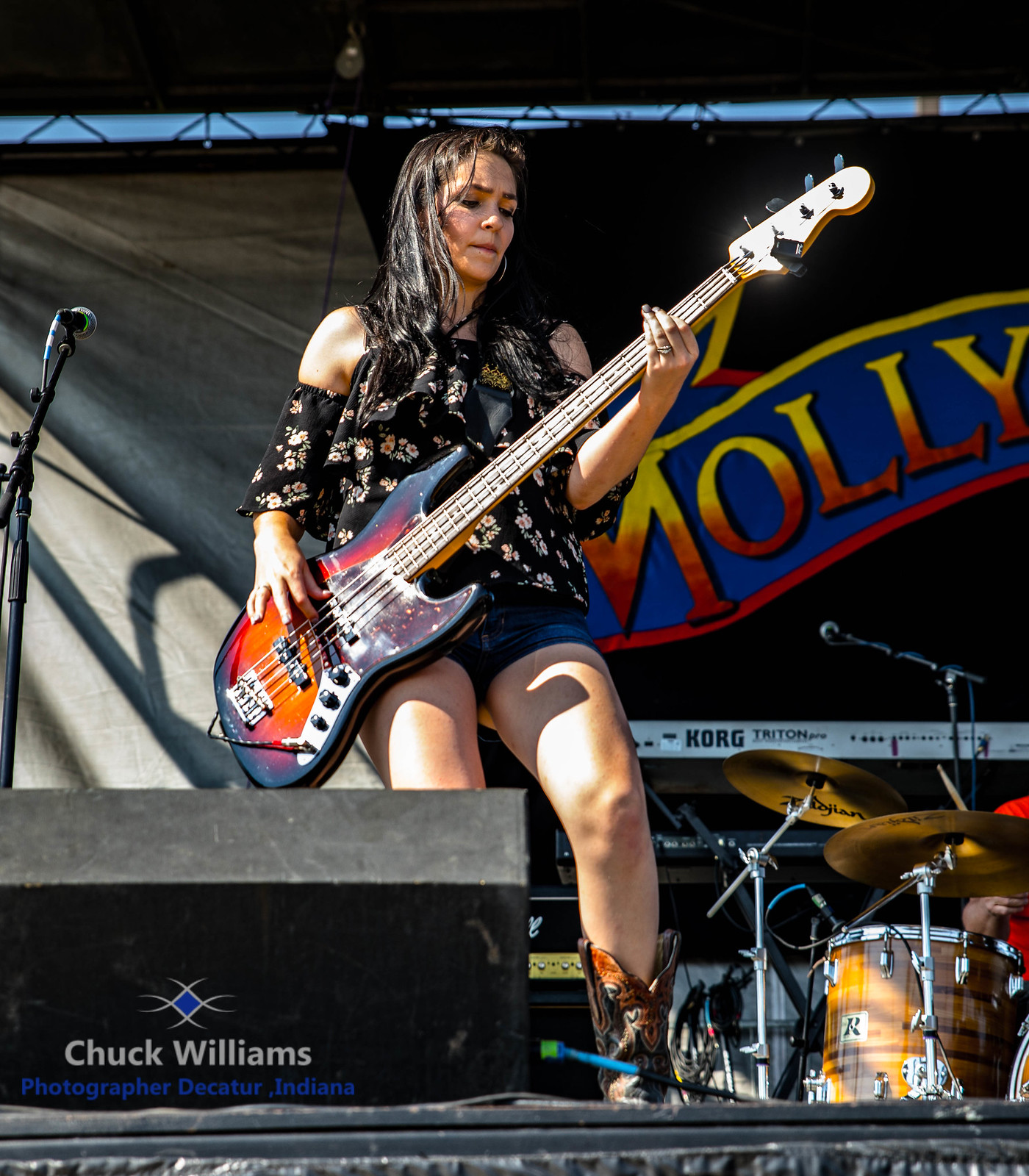The image is a square-format, color photograph of a female rock musician, captured during an outdoor concert in the daytime. The perspective is from the ground, looking up at the stage. The musician, dressed in a black floral blouse with cut-out shoulders, denim shorts, and black cowboy boots, is playing a Fender Precision Bass. She has long, dark hair and is standing in a dynamic pose with her left leg forward, gripping the neck of the bass with her left hand.

To her left, there's a microphone positioned for vocals, and she is flanked by a small speaker. Behind her, a drum kit and a Marshall amplifier are visible, along with various other stage equipment including a Korg keyboard. The backdrop features a black tarp and a banner with the word "Molly," likely indicating the band's name, possibly Molly Hatchet. The photograph shows a sliver of blue sky above the stage and is bathed in sunlight, highlighting the musician. On the lower left corner of the image, the logo reads "Chuck Williams, photographer, Decatur, Indiana," identifying the photographer.

The overall scene captures an energetic moment at an outdoor rock concert, with the vibrant colors of the stage equipment and the musician's attire contrasting against the natural brightness of the day.